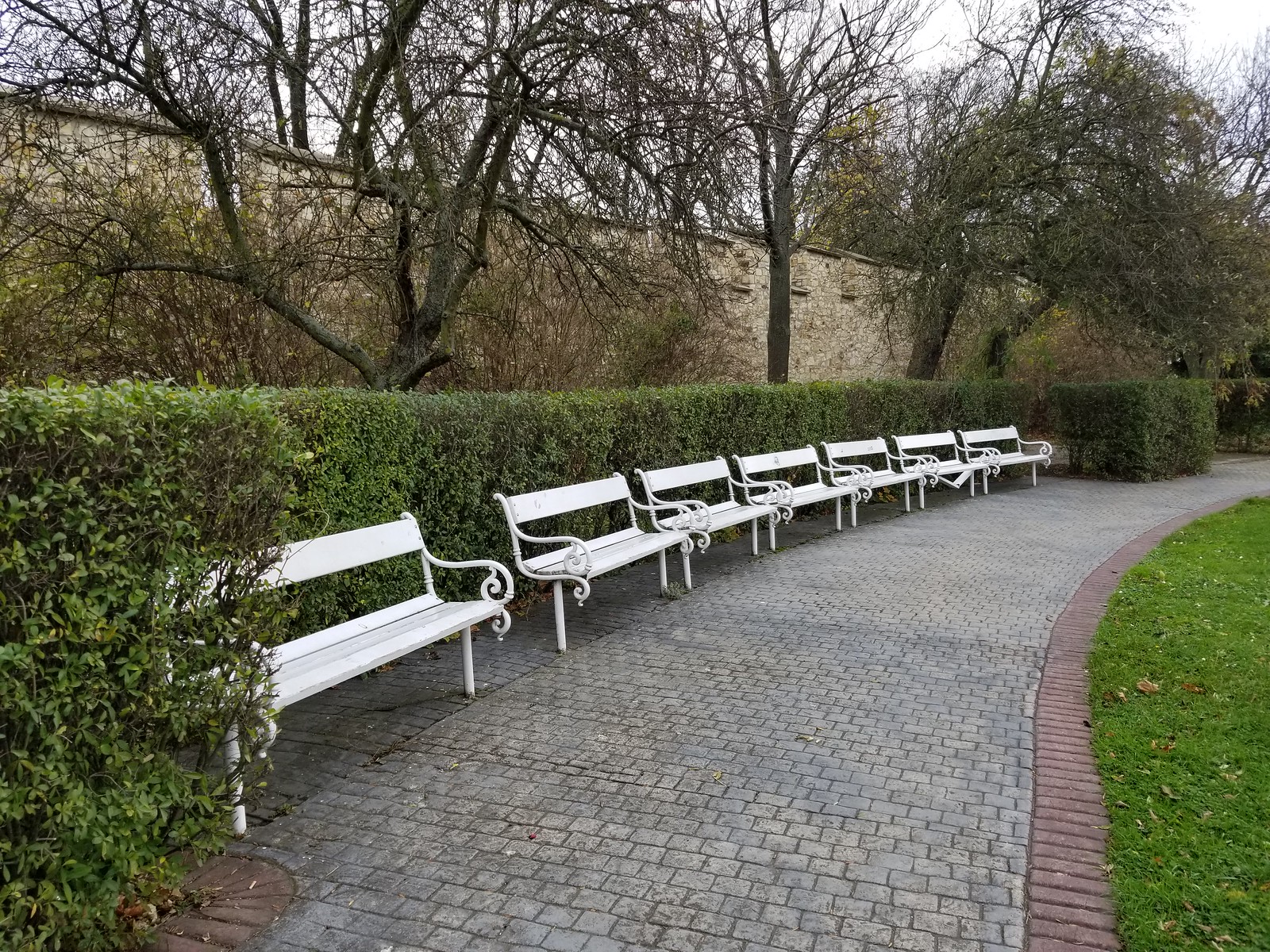This is a detailed color photograph of a peaceful park scene, characterized by a wide, paved walkway constructed with gray cobblestone-like bricks. The walkway is edged on one side with vertical red bricks and on the other by a neatly clipped green lawn. The walkway is flanked on the left by a meticulously trimmed rectangular green hedge. In front of the hedge, there is a row of seven white park benches, each featuring curved ironwork armrests painted white, and composed of four horizontal slats for the seat with an additional slat forming the backrest. Behind the hedge, numerous deciduous trees, mostly bare of leaves, extend upwards. These trees are in front of a large gray stone wall that resembles a castle's perimeter, though no castle is visible in the image. The wall stretches across the background, partially obscured by the bare branches of the trees, with hints of the skyline peeking through the upper branches. The overall composition captures a serene moment in the park, with all elements in sharp focus.